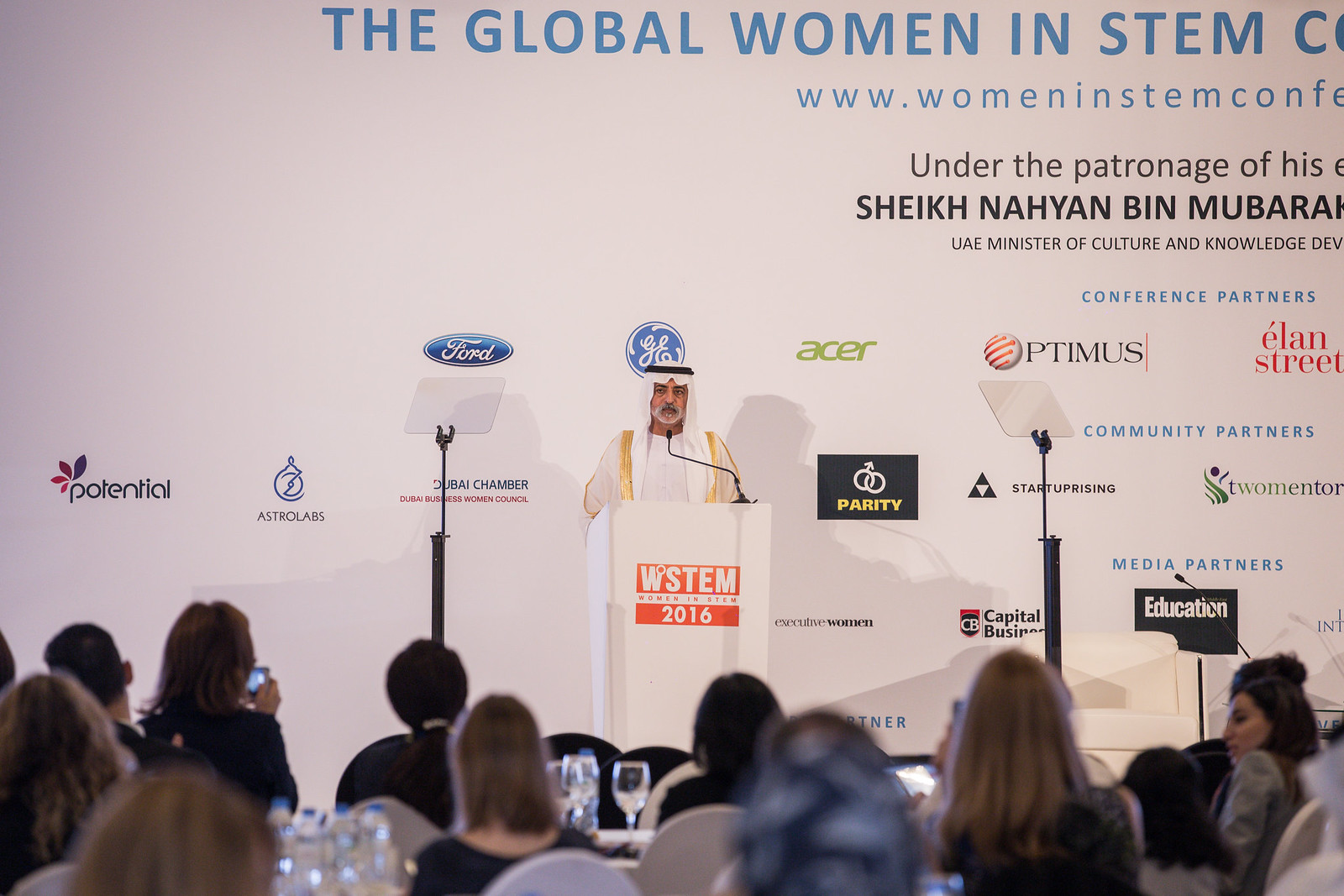The image depicts a man with gray facial hair, wearing a traditional white headdress and a black headband, speaking at a seminar from a white lectern. The lectern features an orange background with white text that reads "WSTEM 2016." He is dressed in a white robe and stands behind a microphone mounted on the lectern. The audience, facing him, consists of several people, whose heads are visible in the foreground. Flanking the lectern are additional microphone stands. The backdrop is a white wall adorned with various corporate logos, including Ford, GE, Acer, and Optimus. At the top, in blue text, partially visible, it reads "The Global Women in STEM," followed by the truncated URL "www.womeninstemconf…". Beneath this is black text that states, "Under the patronage of His Excellency Sheikh Nahayan Mabarak Al Nahayan, UAE Minister of Culture and Knowledge Development."